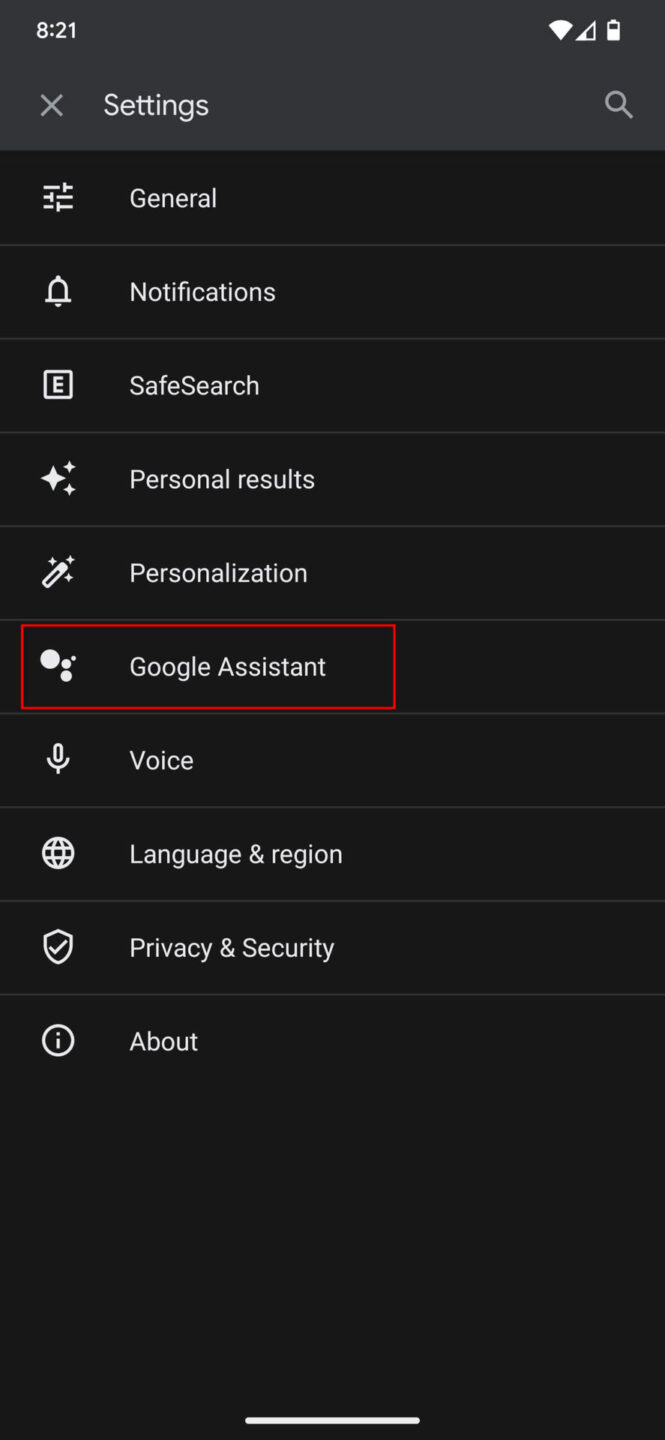Screenshot of a mobile phone displaying the settings menu in high detail. The image is a vertical rectangle with a primarily black background. At the top, a slightly lighter black bar contains the time "8:21," alongside icons for signal strength, battery life, and a triangle-shaped symbol. The word "Settings" is also displayed in this top bar.

Below, the settings menu lists various options in white text, each accompanied by a distinct icon on the left. The listed options include:
- General Notifications (bell icon)
- Safe Search (square with an 'E' icon)
- Personal Results
- Personalization
- Google Assistant
- Voice
- Language and Region
- Privacy and Security
- About

Notably, the "Google Assistant" option is highlighted with a red border around both its icon and text, suggesting it has been selected or tapped by the user. The screenshot does not provide any information to identify the phone model or operating system.